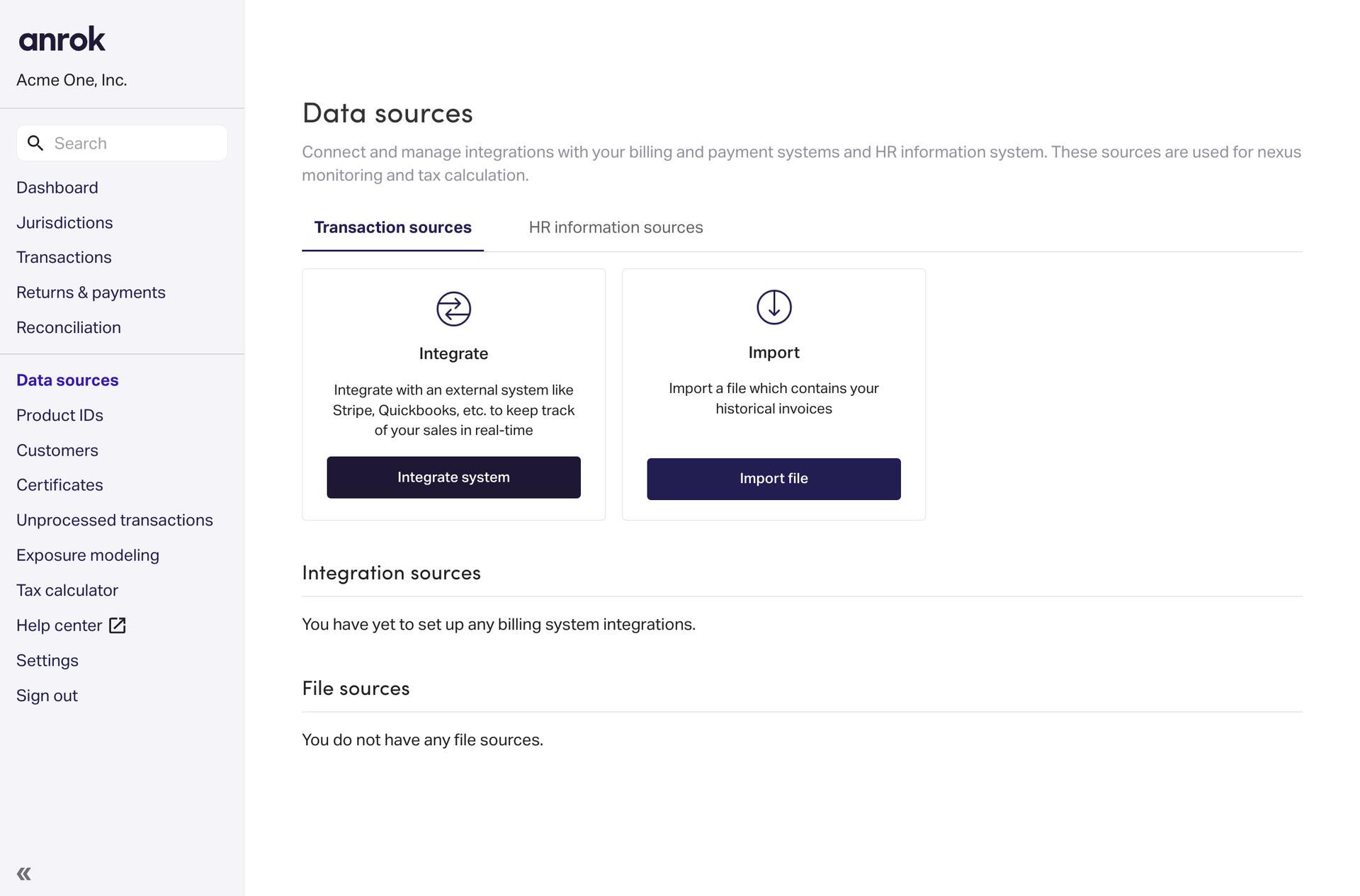The image is a detailed snapshot from a webpage featuring the interface of a software platform. On the left side, there's a sidebar with a subtle lavender-purple gradient that borders on gray. At the top of the sidebar, the heading "ANROK" is prominently displayed, followed by "Acme One Incorporated." Below these titles, a search bar is present, and beneath it, the navigation menu lists several options: Dashboard, Jurisdictions, Transactions, Returns and Payments, and Reconciliation. A faint gray line demarcates the next section with additional options: Data Sources, Product IDs, Customers, Certificates, Unprocessed Transactions, Exposure, Modeling, Tax Calculator, Help Center, Settings, and Sign Out. The "Data Sources" option is highlighted in purple, indicating it is selected. 

In the main content area, the heading "Data Sources" is prominently featured. The section provides a brief description: "Connect and manage integrations with your billing and payment systems and HR information systems. These sources are used for nexus monitoring and tax collection." Below this description, two clickable rectangular buttons are visible, labeled "Integrate" and "Import."